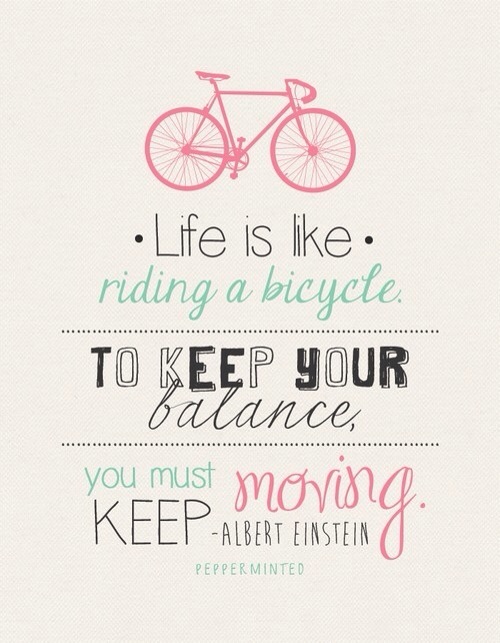The image features a motivational quote against a light tan backdrop. At the top center, there's an icon of a pink bicycle. Beneath the bicycle, the text reads: "Life is like", in black font, and "riding a bicycle" in green italics. Below this, in a mix of black and white stenciled letters, it continues with "To keep your balance, you must keep moving." The words "you must" are in green, "moving" is in pink, and "keep" and "Albert Einstein" are in black. The quote is attributed to Albert Einstein, with a small note at the bottom that says "Pepperminted" in green mint font. The entire layout suggests it's a motivational poster, likely shared on social media for its inspirational message.